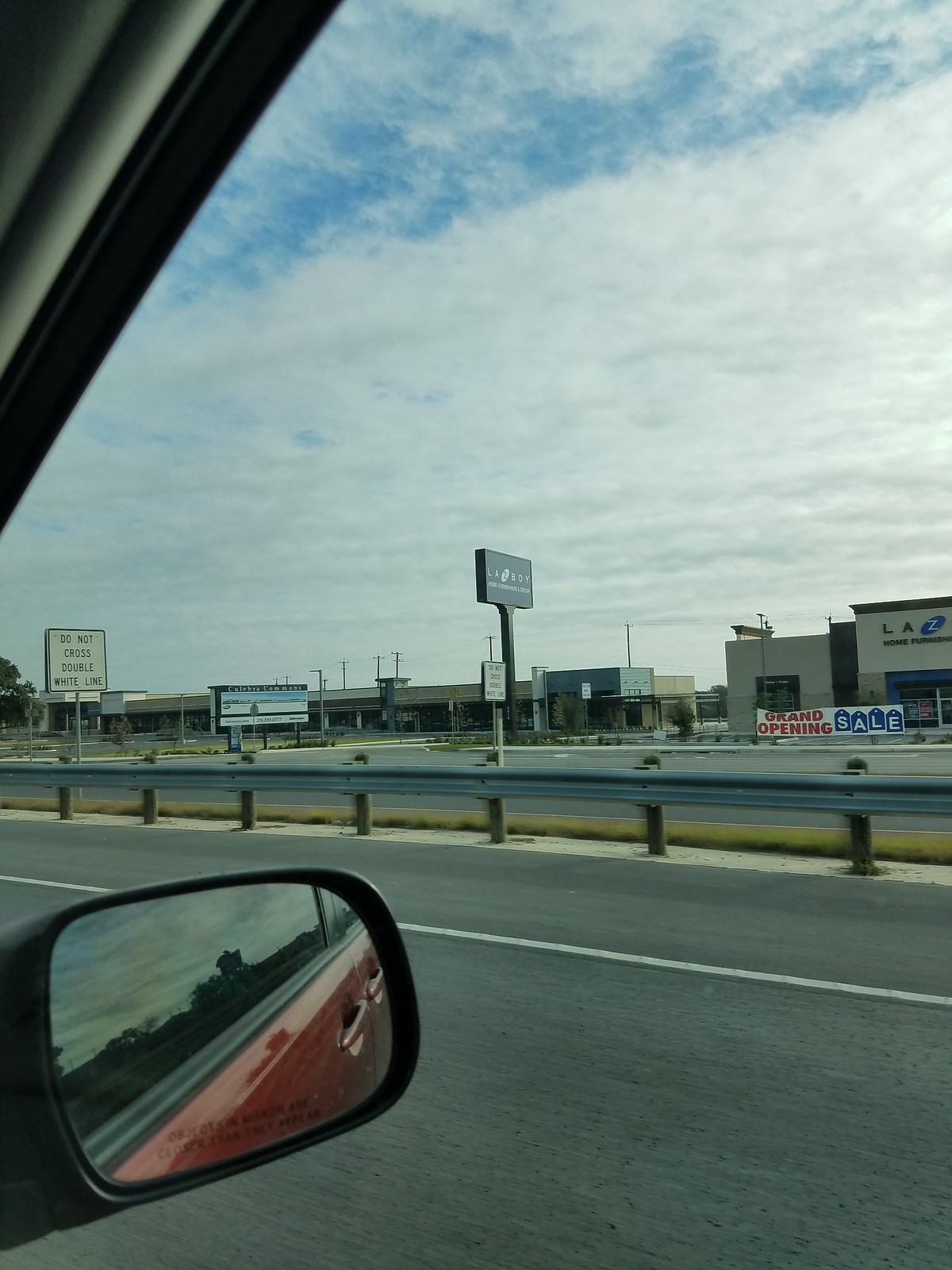This color photograph captures a roadside scene, seemingly shot from inside a vehicle. In the bottom left corner, part of the side mirror is visible, reflecting a red-hued image and part of the roadside. The top corner of the image reveals a section of the vehicle frame, which appears slightly underexposed or filtered with a dark tint.

The road, seen through the vehicle window on the right, is grey with a continuous white line running parallel to its direction. Adjacent to the road is a grassy ridge, accompanied by a horizontal grey metal barrier supported by posts.

In the background, there are several street signs: a prominent white sign with black text on the left, a thinner, taller sign that is difficult to discern, and another smaller sign. Beyond these signs, a row of buildings extends across the scene, escalating in height as they move to the right.

The sky is predominantly overcast, but patches of blue peek through at the top, adding a touch of color to an otherwise cloudy day.